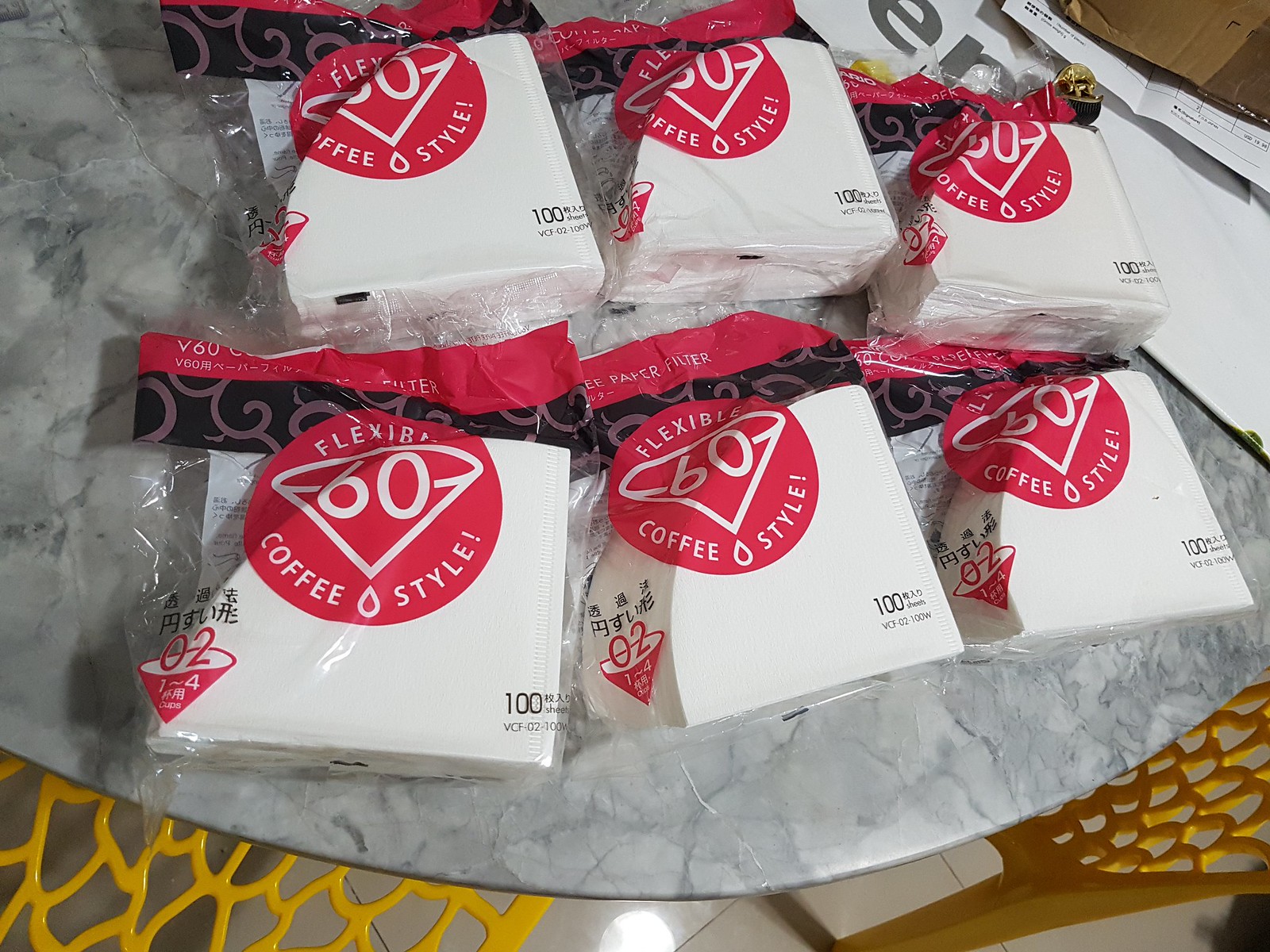In this detailed color photograph, we see six packages of cone-shaped coffee filters, each containing 100 sheets, arranged in two rows on a circular, gray marbled granite table. The packaging is predominantly white with red accents, featuring a red circle with the white text "Flexible Coffee Style" and an icon resembling an upside-down pyramid with the number "60" inside, and a teardrop shape beneath. The model number "VCF-02-100W" and "100 per bag" are also clearly visible. Surrounding the table are wooden chairs, and some papers can be seen in the background, enhancing the domestic setting. The photograph is taken from above, offering a clear, unobstructed view of the arranged packages.